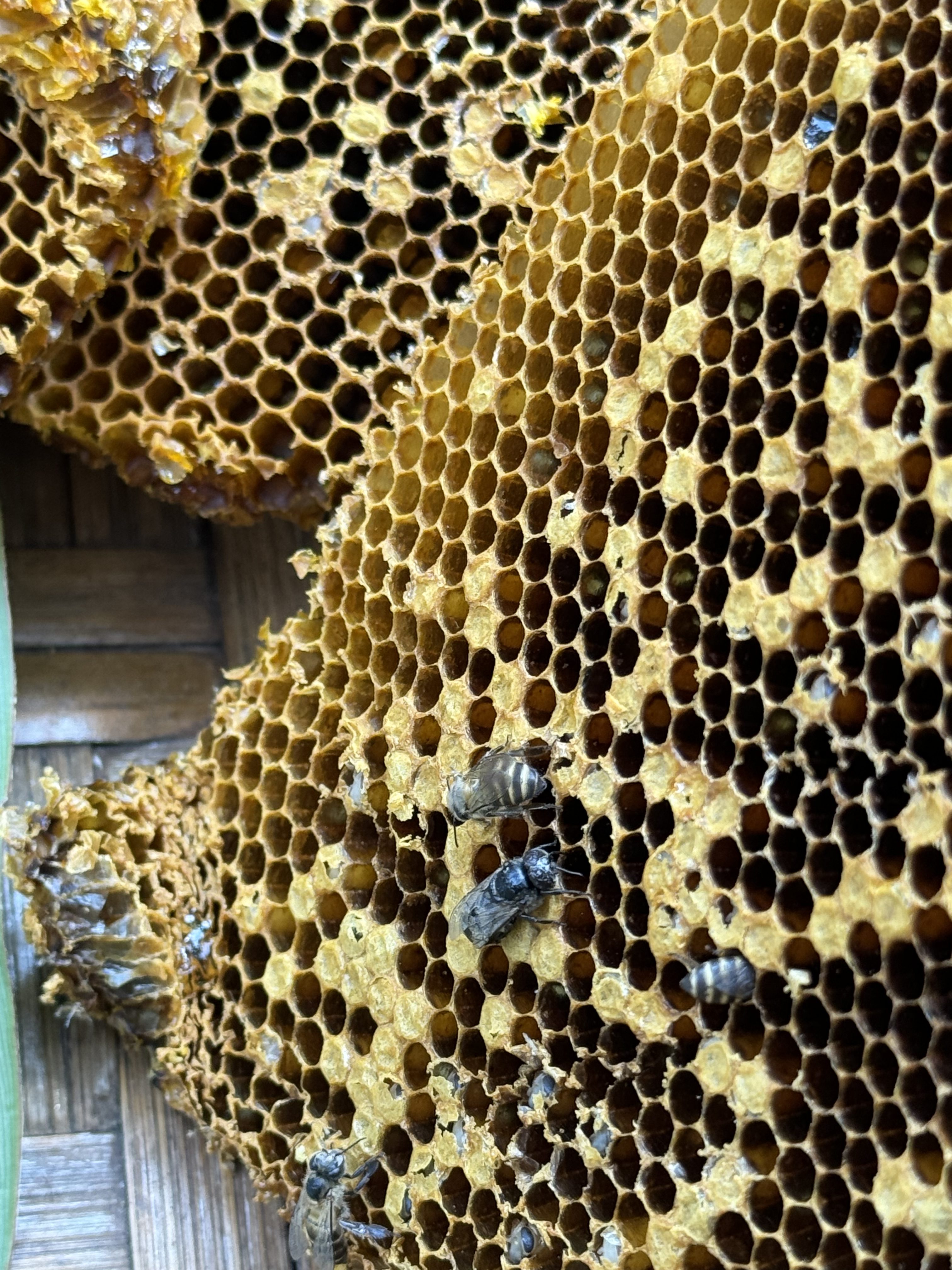This detailed photograph captures an exceptionally large honeycomb with distinctive features. Notably, two sections of honeycomb are visible, set on a tiled floor. The honeycomb, with its characteristic yellow pattern, appears slightly ravaged as if recently removed from its original setting. Despite its relocation, a scattering of bees remains actively crawling around, tending to their cells. The bees are notably darker than typical honey bees, almost black in color, and are not as numerous as usually seen. In the background, wood slats are faintly visible, adding an intriguing element to the scene. The image evokes curiosity about the honeycomb’s origins and the story behind its unusual placement.